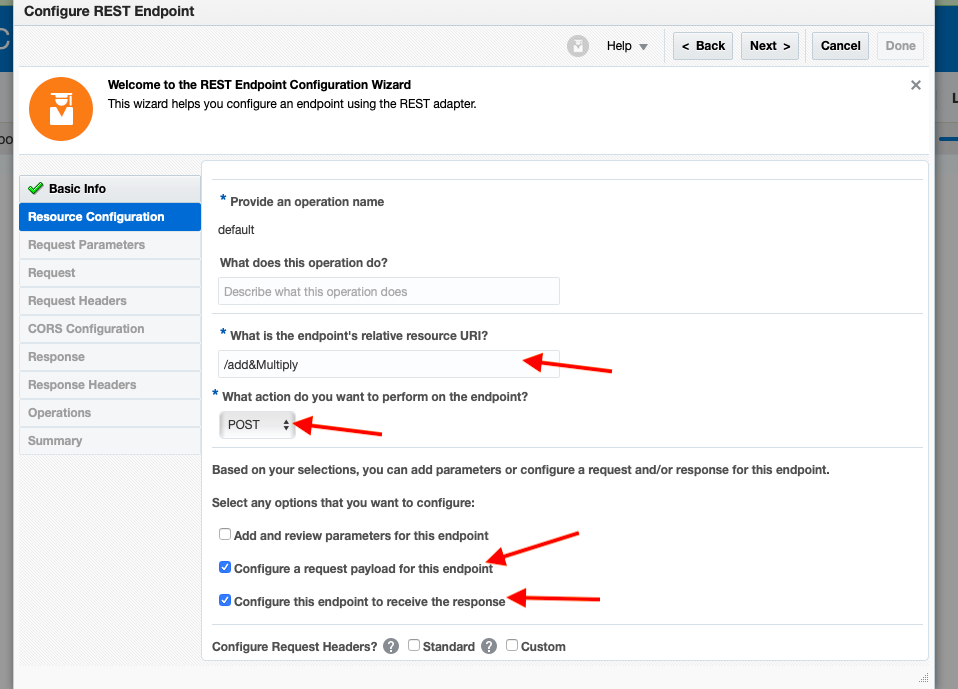Here is a cleaned-up and detailed caption for the described image:

---

The image displays a website interface for configuring REST endpoints. At the top left corner, bold black text reads "Configure REST Endpoint." Directly below this header, there is a search bar. To the right of the search bar, there's a help icon with a downward-facing arrow, and further to the right are several navigation buttons: back, next, cancel, and a "Done" button which is greyed out.

Beneath this, towards the left, there is an icon—a white outline of a person wearing a graduation cap set against an orange circle. Next to this icon, bold black text states, "Welcome to the REST Endpoint Configuration Wizard." Below this welcome message, another line of text explains, "The wizard helps you configure an endpoint using the REST adapter."

On the left-hand side, a vertical menu lists steps for configuration. The first item, "Basic Info," marked with a green checkmark, is in bold black letters. The second item, "Resource Configuration," is highlighted in blue with white text, indicating the current step. Subsequent items— "Request Parameters," "Request," "Request Header," "CORS Configuration," "Response," "Response Headers," "Operations," and "Summary"—are all in grey text, denoting steps yet to be completed.

To the right of this vertical menu, a detailed pop-out menu is displayed under "Resource Configuration." This menu asks for input with various prompts:
1. "Provide an operation name," with the default text "default" underneath.
2. "What does this operation do?" followed by an empty search button.
3. "What is the endpoint's relative resource URI?" accompanied by a text input box containing "/ADD&MULTIPLY." A prominent red arrow points towards this text box.
4. "What action do you want to perform on the endpoint?" listed with a "POST" button featuring an up-and-down arrow inside of it, and a bold red left-facing arrow beside it.

The overall interface is designed to guide users through the process of configuring a REST endpoint, clearly laying out each step and providing input fields for the required information.

---